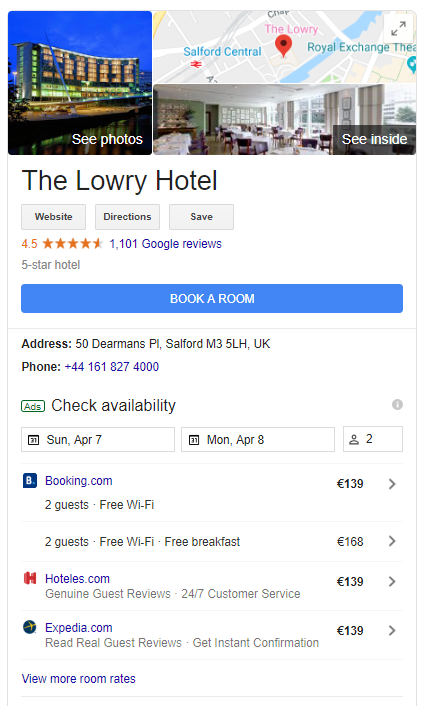The image features a comprehensive informational display against a white background. At the top left corner, there is a stunning photograph of a large hotel under a clear blue sky, captioned "See Photos." Adjacent to this, on the top right, is a map next to an interior snapshot of the hotel lobby with a button labeled "See Inside."

Positioned central to the image is the name "The Lowry Hotel" prominently displayed with options for "Website," "Directions," and "Save." It is rated 4.5 stars based on 1,101 Google reviews and is designated a five-star hotel. Below this, a blue box prompts users to "Book a Room," providing the hotel's address at 50 Dearman's Place, Salford, M35LH, UK, and a contact phone number: +44-161-827-4000. A small green box indicates "Ads."

To the right, there is a grey circle with an “i” enclosed, followed by dropdown menus for selecting dates, including Sunday, April 7th, and Monday, April 8th, as well as an option for indicating two guests. Beneath these features, a blue box links to "Booking.com," listing room rates at 139 Euros for two guests with free Wi-Fi and 168 Euros for two guests with free Wi-Fi and breakfast. Each rate is accompanied by a right arrow.

Additional room rates from various booking platforms are displayed: 
- "Hotels.com," marked with a small red "H," promotes genuine guest reviews and 24/7 customer service, pricing at 139 Euros with a right arrow.
- "Expedia.com," indicated by a blue circle with a yellow cross, offers instant confirmation and real guest reviews, also at 139 Euros with a right arrow.

At the bottom, there is an option to "View More Room Rates."